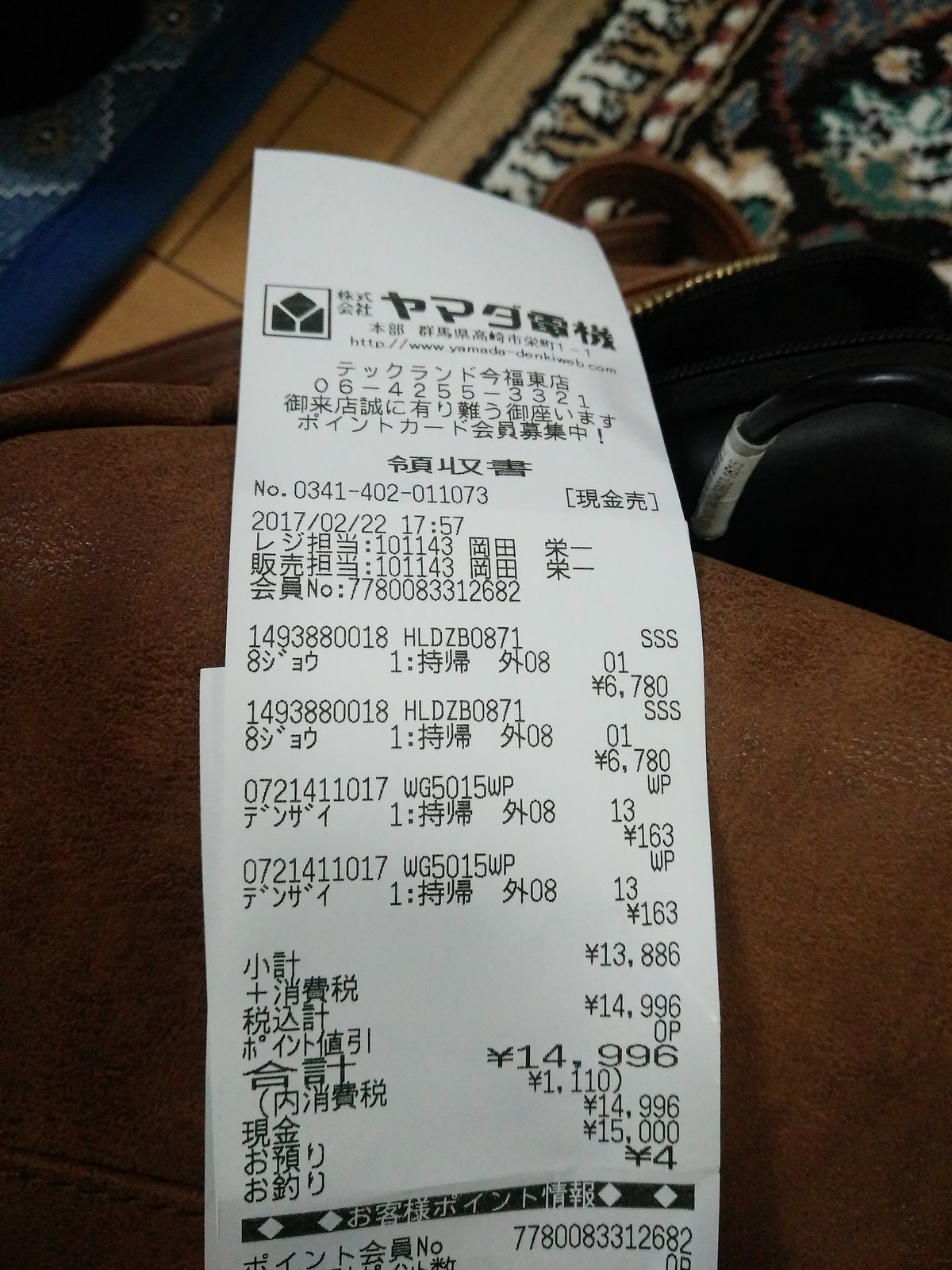The image features a non-English receipt placed on a brown blanket. The receipt displays English numerals, with the total amount of 14.996 emphasized in larger font at the bottom. A black logo composed of three shapes is situated at the top left corner of the receipt. Surrounding the receipt, a black purse rests at the front, while a multicolored rug—comprising tan, black, blue, and red hues—spreads out beneath it. Additionally, a small section of flooring is visible on the left, accompanied by a blue rug in the top left corner.